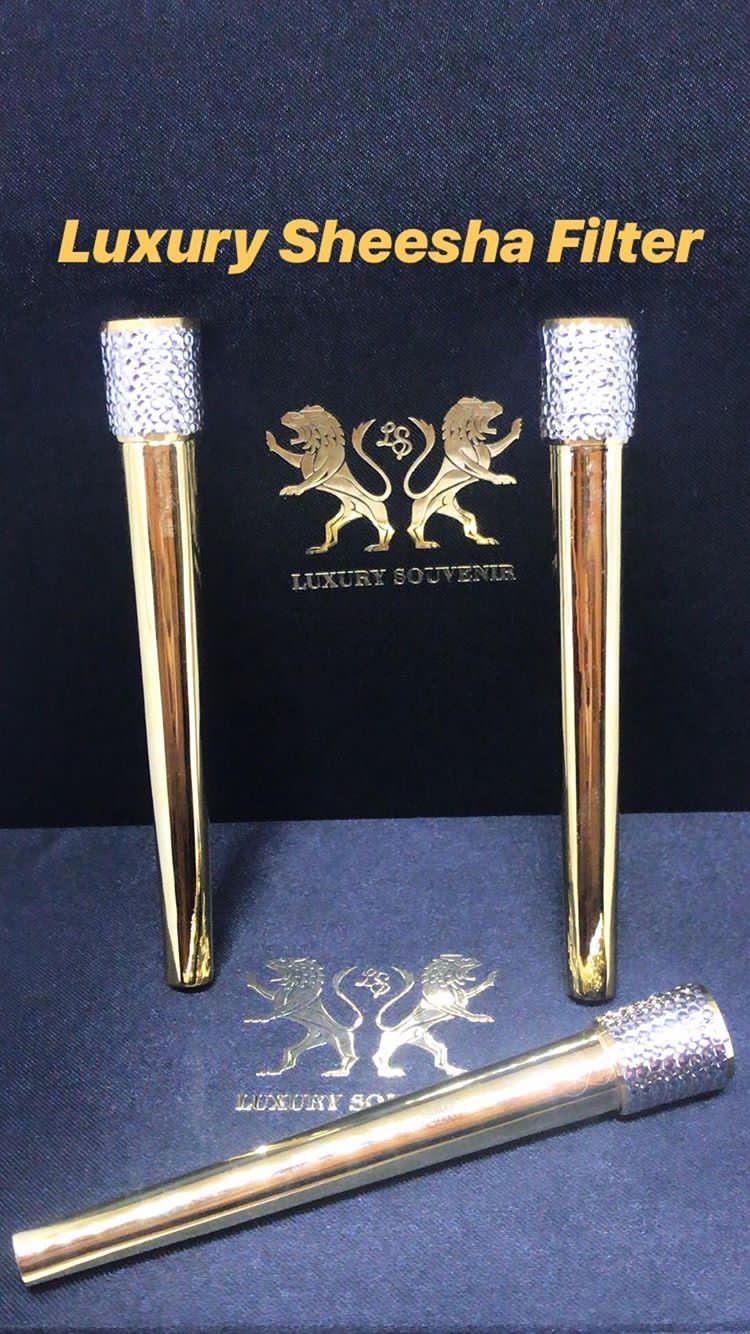In this intricately detailed photograph, we see three opulent shisha filters presented elegantly. Each filter is a cylindrical gold structure with a silvery, diamond-like adornment at the top. The first two filters stand upright, leaning against a dark blue box or wall, while the third filter lies horizontally in front of them, adjacent but slightly separated from the others. Dominating the center of the scene is a luxurious logo featuring two golden lions, exquisitely crafted in silhouette form, facing opposite directions. Their tails curve around to encircle the scripted initials "LS" which stand for Luxury Souvenir, denoted below in lavish golden text. The entire arrangement exudes an aura of sophistication and refinement, with attention to every detail enhancing the sense of luxury.